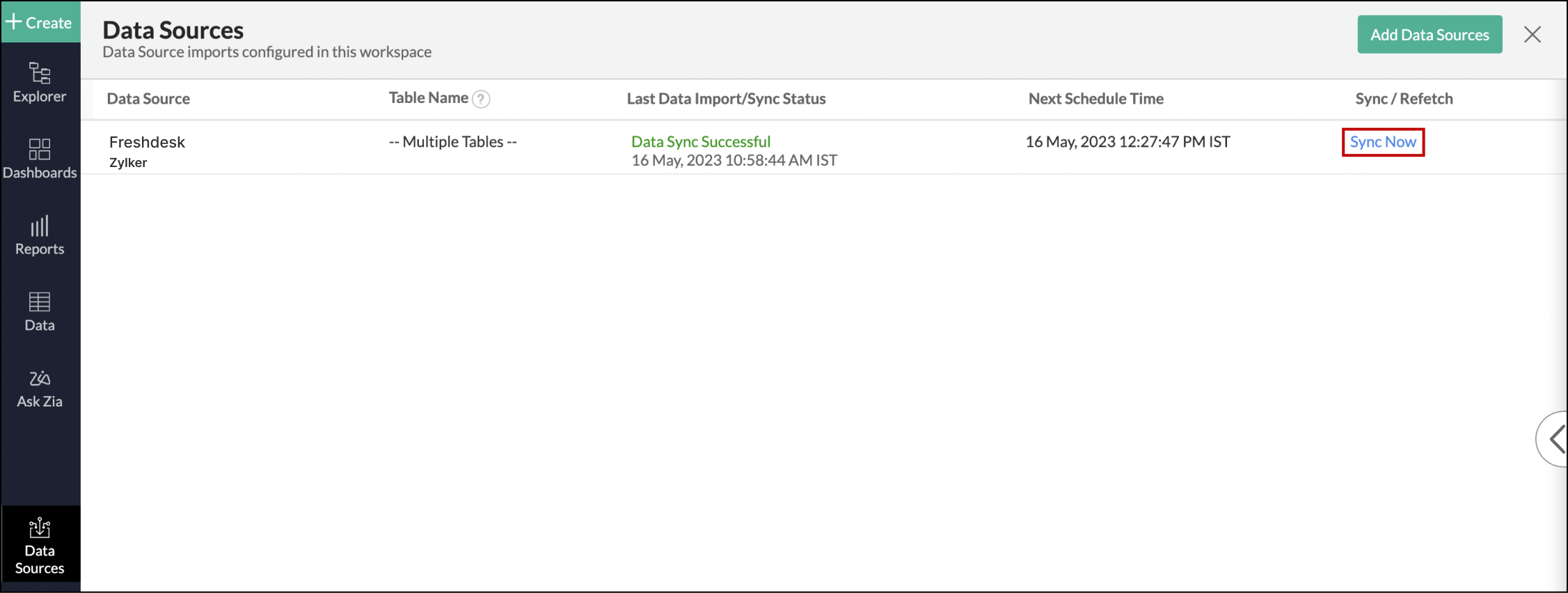In the image, the interface is divided into two primary sections. On the left side, there is a vertical menu with a navy blue background. The menu items are listed sequentially from top to bottom. The top-most button is green and labeled "Create" located in the top-left corner. Below this, the menu options with a navy background are listed as: "Explorer," "Dashboard Reports," "Data," "Ask Zia," and the last option, which has a black background, is "Data Sources."

On the right side of the interface, the background is white. At the top, it prominently displays the heading "Data Sources." Underneath, it reads "Data Source Imports Configured in This Workplace." The main section features a table with five columns labeled: "Data Source," "Table Name," "Last Data Import/Sync Status," "Next Scheduled Time," and "Sync/Refresh."

Within the table, there is one data source entry:

- **Data Source**: Freshdesk, Zalka
- **Table Name**: Multiple tables
- **Last Data Import/Sync Status**: Data sync successfully (written in green)
- **Date**: May 16, 2023, 10:58:44 AM IST
- **Next Scheduled Time**: May 16, 2023, 12:27:47 PM IST
- **Sync/Refresh**: Sync Now (button is blue with a red outline)

In the top-right corner of the white section, there is a green button labeled "Add Data Sources."